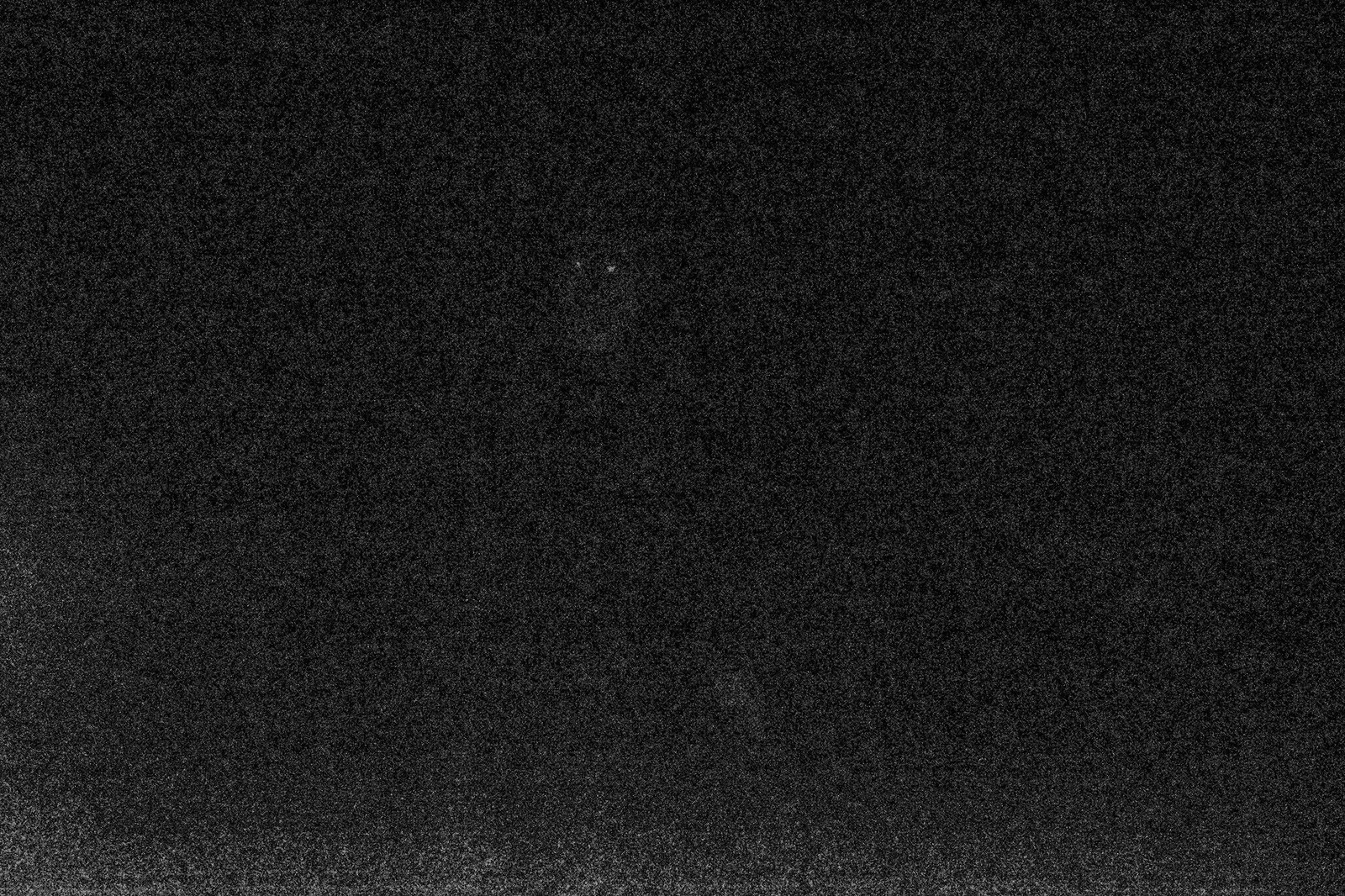The image depicts a grainy and blurry photograph dominated by black and dark gray tones, resembling static from an old, fuzzy VHS tape. The overall texture is very coarse and washed out, creating a noise-filled visual. In the upper center portion of the rectangular frame, there is a vague, whitish shape that might be interpreted as a face. Within this face-like shape, two clear white dots stand out, resembling eyes, with slightly separated gray above them suggesting faint eyebrows. The ghostly figure in the center could possibly represent a man with crossed arms, but the details are very indistinct. Additional smudges of gray can be found towards the bottom of the image and sporadically on the right and left sides, but the majority of the photograph remains engulfed in darkness.